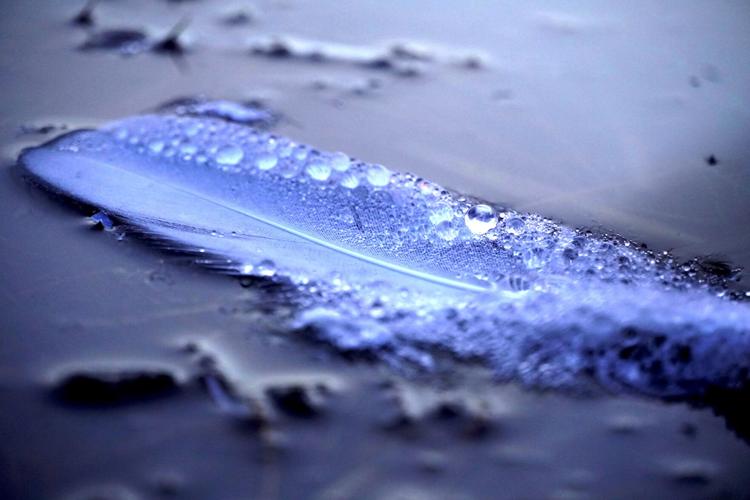The image is a very detailed, close-up photograph of a bright, vibrant blue feather, possibly with a purplish tint, lying on a somewhat irregular surface. The feather, which dominates the center of the image, is adorned with glistening water droplets that look almost like tiny glass spheres due to their perfectly round and translucent nature. The water droplets are primarily clustered along the central vein, which runs from a thicker base on the right to a thinner tip on the left. The feather's fibers are wispily edged, providing a beautiful contrast to the smooth, shiny droplets. The surface beneath the feather appears to be a muted blue or possibly wet sand-like material, blurred and lacking distinct definition. The background has a gray to almost black coloring and remains largely out of focus, enhancing the feather's prominence and the fine details of the water droplets above it. There are subtle reflections of light, especially on the water bubbles, adding a dynamic, almost shimmering quality to the feather's appearance. Overall, the image captures an exquisite and intricate view of nature, highlighting each delicate component of the feather and the water droplets it holds.